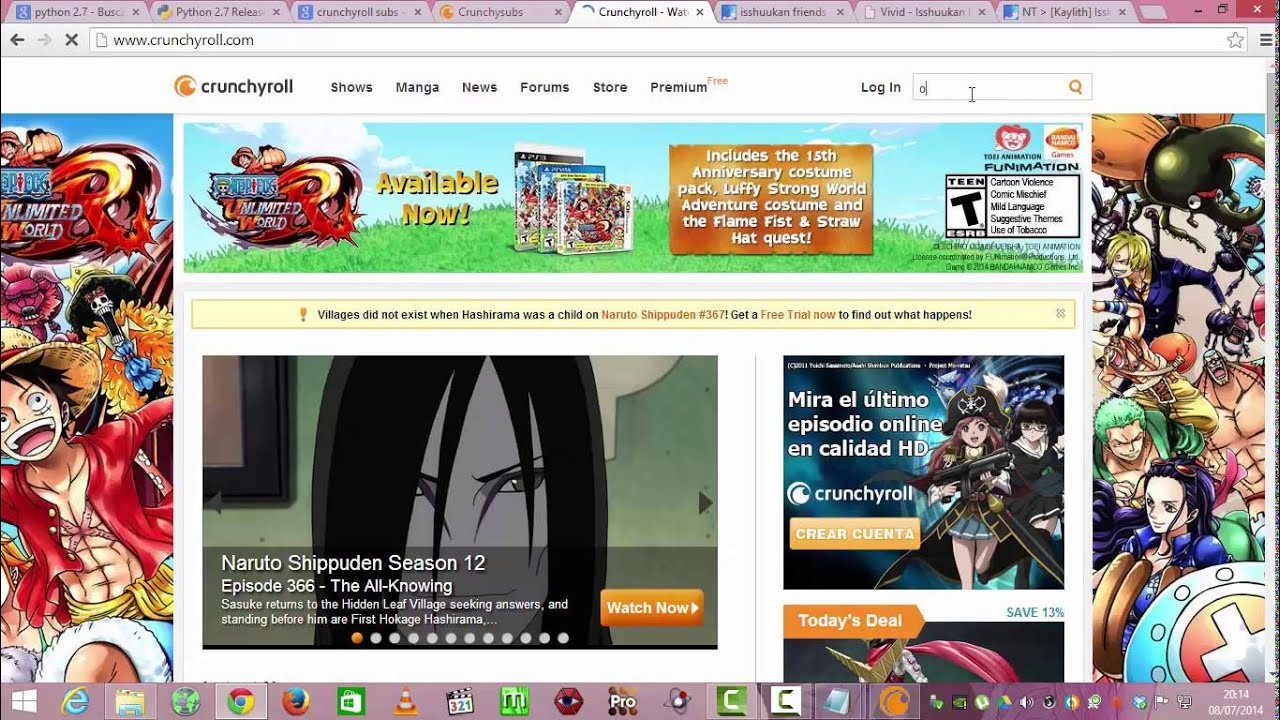This image is a screenshot from the website Crunchyroll.com, showcasing a page that appears to promote a video game. The main background features various video game characters with diverse hair colors, including green, orange, and yellow. These characters are dressed in different styles of clothing, with some male figures displaying their chests prominently. 

At the top of the screen, there are several navigation options including Shows, Manga, News, Forums, Store, and Premium, along with a login section. The page highlights a special offer labeled "Available Now," which includes the "15th Anniversary Costume Pack," the "Luffy Strong World Adventure Costume," and the "Flame Fist and Straw Hat Quest." The game is rated "T" for Teen, as indicated by the rating box.

Towards the middle of the screen, there is information about a specific anime series: "Naruto Shippuden Season 12," featuring Episode 366 titled "The Unknowing." Various other UI elements and details are present, enhancing the comprehensive interface of the webpage.